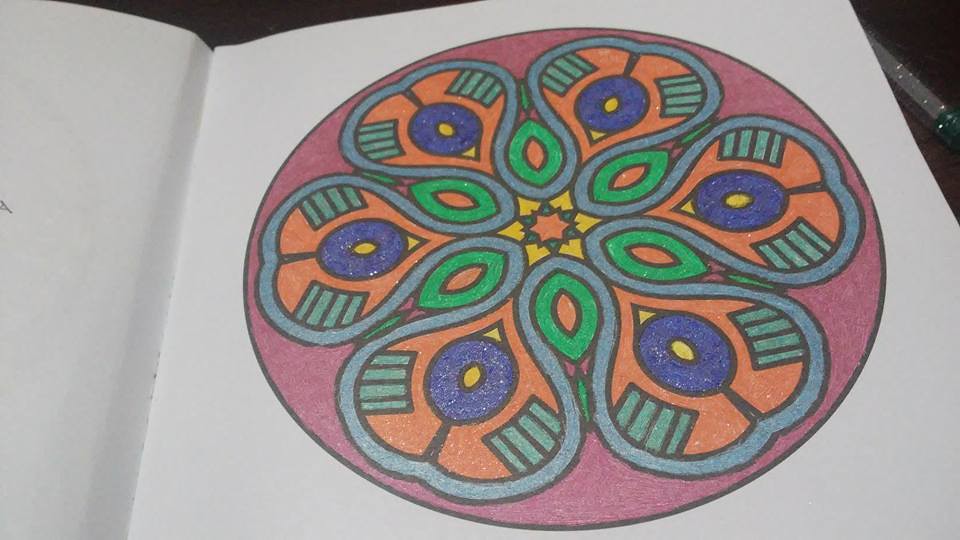A vibrant hand-colored illustration adorns this white sheet of paper. Central to the image is a large, circular, pink background that frames an intricate array of geometric and floral motifs. Within this pink circle, six petal-like shapes - three at the top and three at the bottom - are meticulously rendered in shades of light blue, orange, navy, yellow, green, and black. These petals encircle a core where smaller green petals emerge, drawing the viewer's eye to the center of the composition. At this focal point, a detailed flower blooms, featuring a blend of yellow and orange hues accented with delicate green markings.